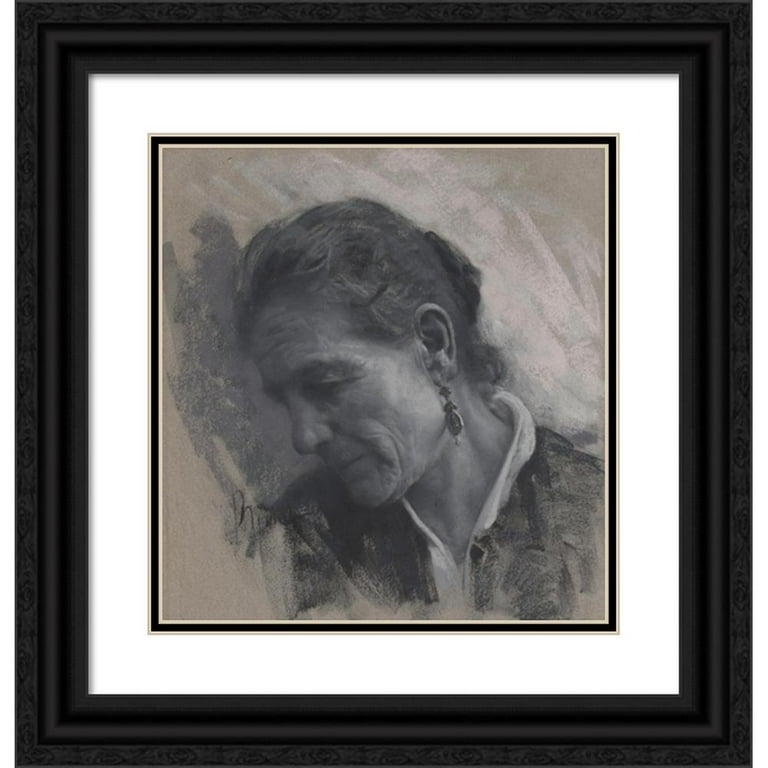This framed artwork, encased in a solid black frame with a white matting and a thin black inner border, portrays an elderly woman rendered in grayscale tones with subtle hints of color, possibly pastels. The subject, appearing to be in her 60s or 70s, has her dark, neatly-tied back hair streaked with wisps of gray. She is seen from the chest upwards, her head tilted downwards to the left, presenting a partial profile view. The woman's face, marked with wrinkles and weariness, carries a solemn, almost grim expression as she looks downwards. She wears a white shirt with a high collar, over which appears to be a dark-colored jacket, and a single dangly earring. The brushstrokes fade into the background, creating a mist-like effect that lends a dreamlike quality to the image.